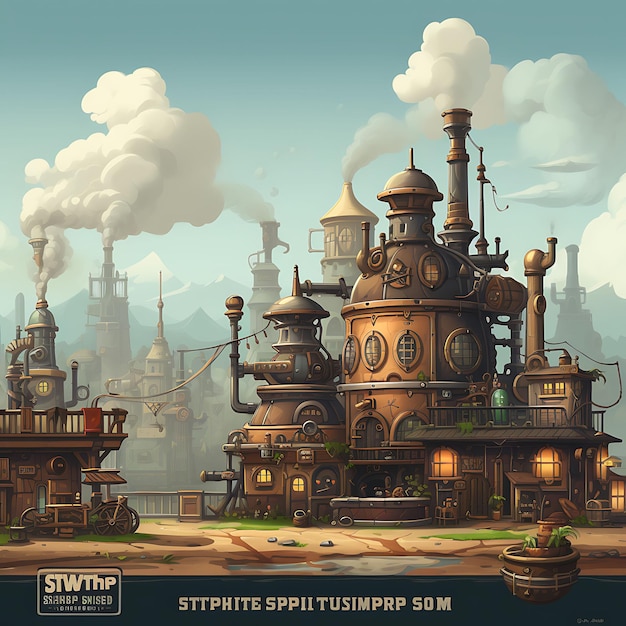The image is a digitally rendered, steampunk-inspired graphic, resembling a copper-colored factory or castle surrounded by similar buildings. The structures, which have a submarine-like feel, feature circular windows with iron grates and numerous pipes emitting steam. In the foreground stands a large, prominent building, with several houses receding into the mountainous background. The scene is accented by a wooden bucket filled with plants, as well as additional greenery adorning some buildings. The color palette includes shades of brown, white, light blue, dark blue, black, green, and copper, with a small puddle adding a touch of blue in the foreground. There is some indecipherable text at the bottom of the image, suggesting it might be generated by AI, with sequences like "S-T-T-P-H-I-T-E-S-P-P-I-I-T-U-S-I-M-P-R-P-50-M" and "S-T-W-T-H-P-G-N-I-S-E-D" appearing on the screen. The overall scene evokes a whimsical, cartoon-like quality reminiscent of a children's movie or storybook setting.